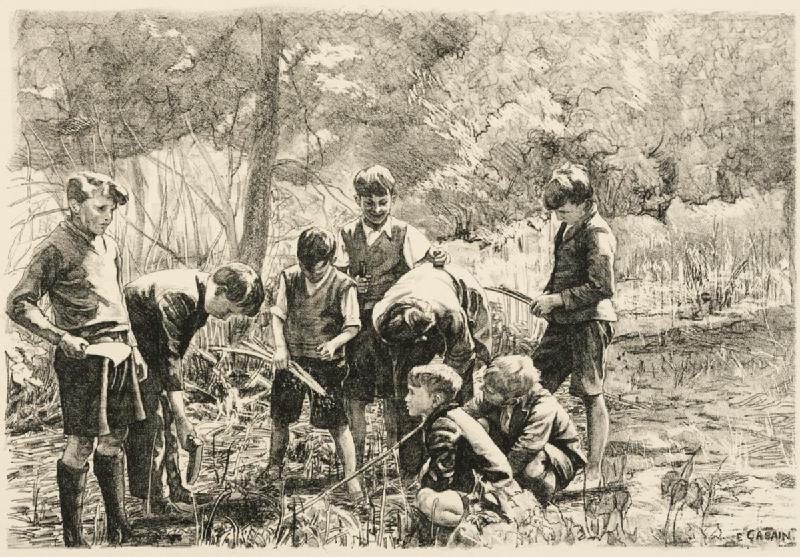This black and white drawing, likely done in charcoal or pencil, vividly captures a group of eight young boys, possibly aged eight to ten, gathered outdoors in a natural setting. The scene features a backdrop of blurred trees, bushes, and what looks like a creek area, with grass shoots sprouting on the ground. The boys are engaged in various activities, with some kneeling and others standing, pointing sticks towards a focal point on the ground that remains indistinct. Their attire includes high socks, shorts, long-sleeved shirts, vests, and waterproof boots, giving a realistic and detailed portrayal. Despite the absence of color, the artwork's detailed rendering conveys a lively depiction of these boys playing, interacting, and smiling in an open field beside the woods, immersed in nature.